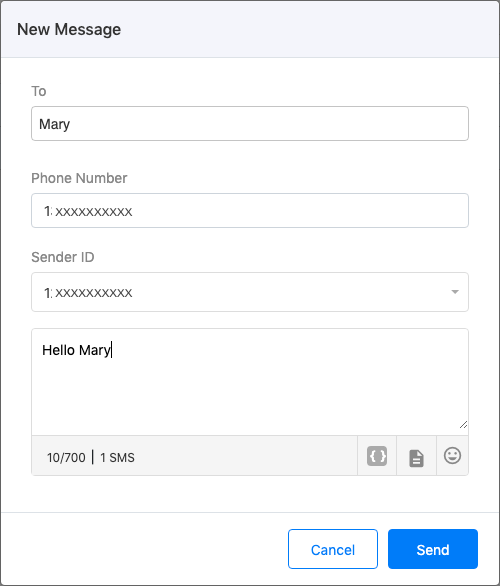The image is a vertically oriented rectangular dialogue box framed by a black border. At the top, a light gray banner spans the width of the image with the text "New Message" prominently displayed. Directly beneath this banner is a field labeled "To," followed by a white input box outlined in black, containing the name "Mary" and a smaller text indicating "Phone number".

Continuing downward, there's another white input box with a black outline, containing the placeholder "1XXXXXXXXXX," signifying a phone number. Below this is a field labeled "Sender ID," accompanied by a similar white box with a placeholder "1XXXXXXXXXX" and a dropdown arrow on the right side.

Further down, there's a larger white text box with a black outline containing the message "Hello, Mary." Underneath this box, a gray border displays the information "10/700, 1 SMS." 

At the bottom of the dialogue box, a thin gray line separates this section from the control options. On the lower right, there are two buttons: a white box with a blue outline labeled "Cancel" in blue text and a blue box labeled "Send" in white text. Several miscellaneous icons are also present in this lower section.